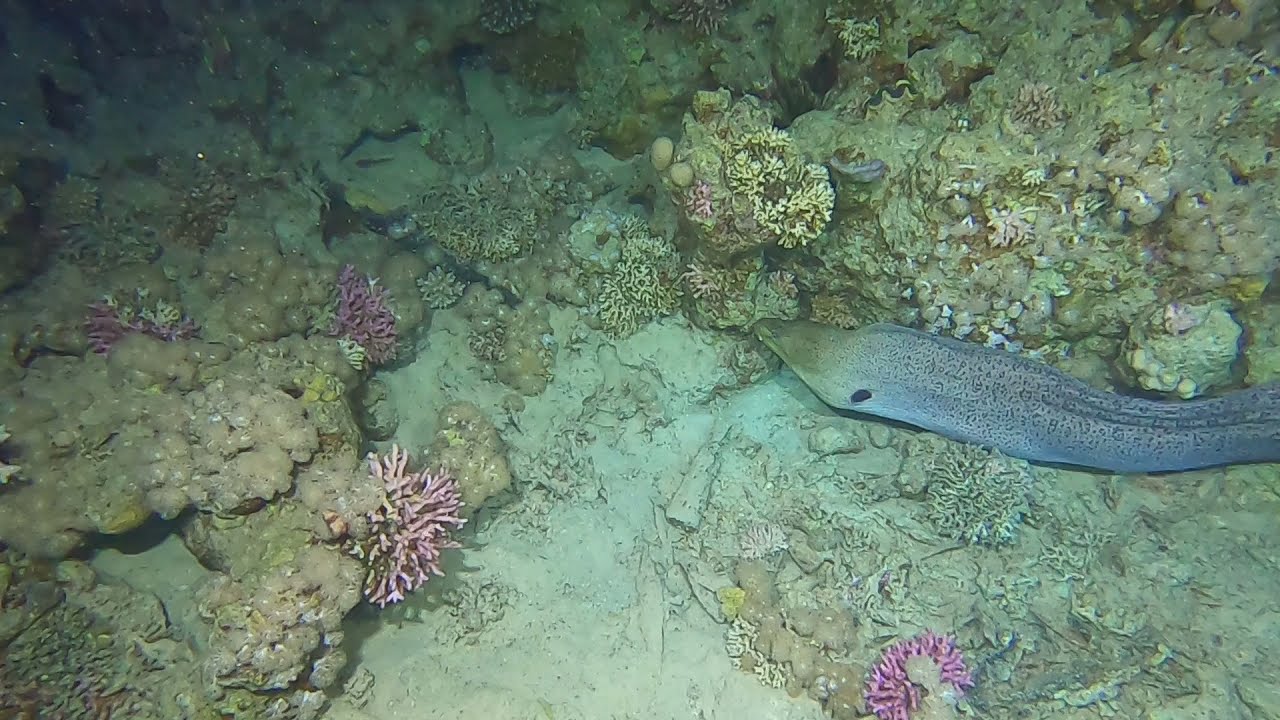This underwater photograph captures a diverse and vibrant ocean floor scene, steeped in a greenish-blue tint that suggests murky water conditions. Dominating the image is a long, flat eel with a blue-grey body, a white underbelly, dark grey spots, and black eyes positioned towards the middle right of the frame, partially out of sight. The ocean floor features patches of white sand interspersed with various types of corals, sea anemones, and other marine plant life. These underwater organisms display a rich palette of colors including pink, purple, green, yellow, and white. Among the corals and anemones, there are also numerous shiny, slimy, beige blobs, roughly the size of baby potatoes, adding to the texture and complexity of the scene. Despite the murky visibility and somewhat unprofessional clarity of the image, the underwater world is thriving with an array of unique and vivid aquatic flora and fauna.